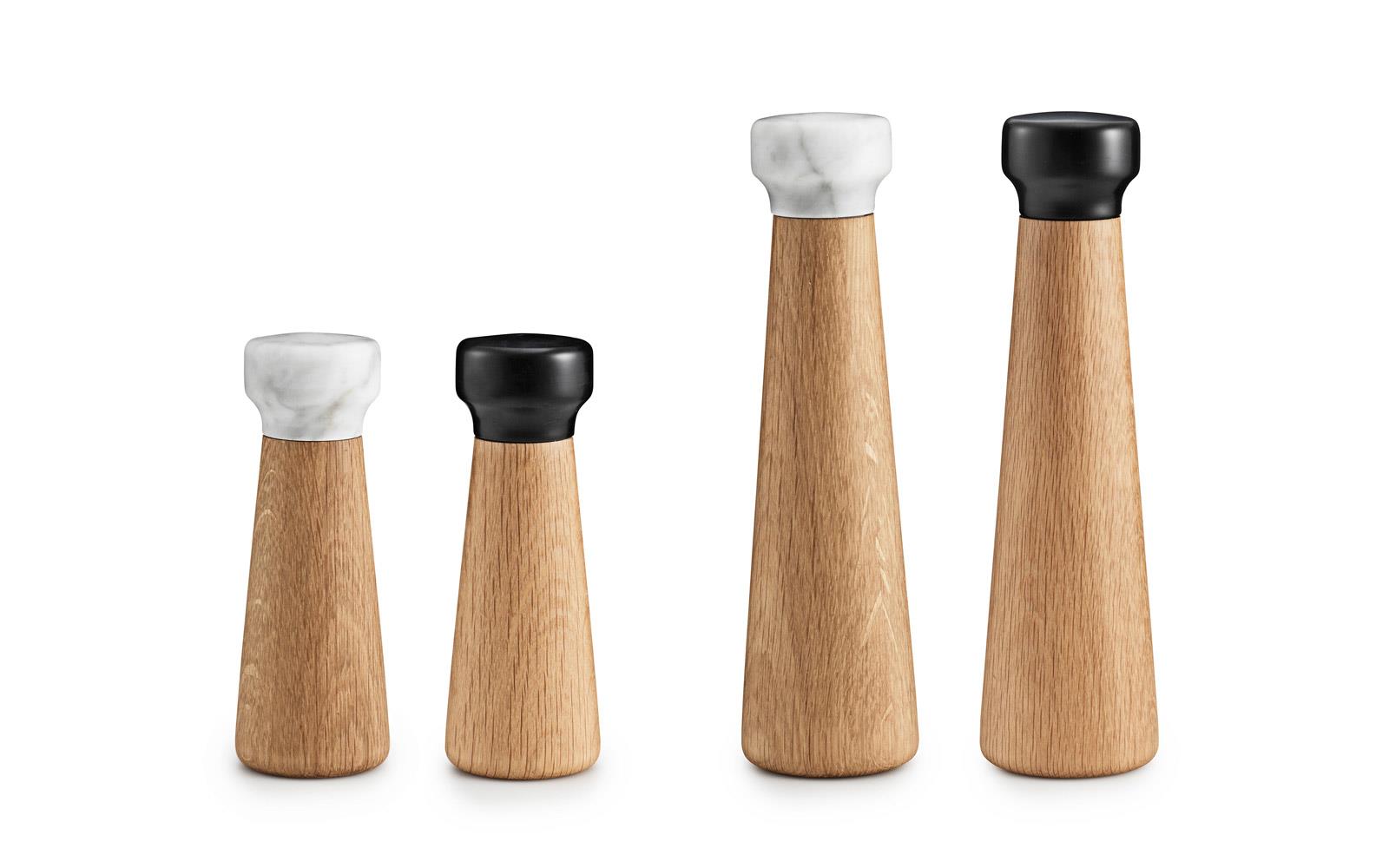This close-up photograph showcases two sets of elegantly designed salt and pepper shakers, each crafted from light brown wood and featuring distinct tops. Both sets, positioned side by side, highlight a contrast in size and color scheme. The shorter set on the left consists of two shakers, approximately 3 inches tall. The shaker on the far left has a lid that is white with gray accents and a flared base, while its companion to the right sports a shiny black lid with a similar flared base. To their right stands a taller pair of shakers, about one-third taller than the shorter set, each mirroring the design of their smaller counterparts. The taller shaker on the left also has a white lid with gray accents, and the one beside it has a black lid. All lids are cylindrical and taper downward. The detailed craftsmanship and uniform wood material lend a cohesive and stylish look, suitable for a product display or an online shopping catalog.